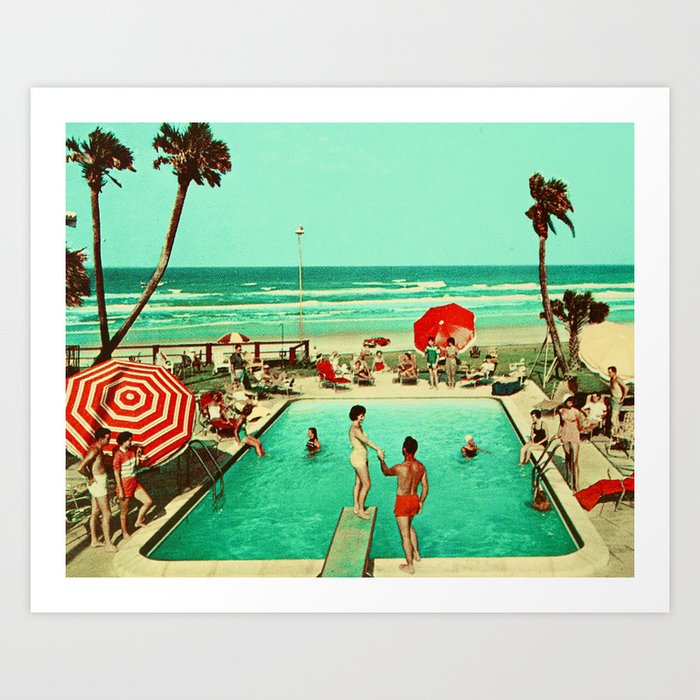This detailed vintage-style painting from around the 1930s to 1960s depicts a lively beachside pool club set right at the sandy edge of the ocean. The focal point is the pool, which is surrounded by numerous adults in various states of undress, primarily enjoying the summer day in their bathing suits. In the very forefront, a woman in a white swimsuit stands gracefully on a diving board, holding hands with a very tan man in red trunks. The pool itself hosts a few swimmers, including a woman wearing a bathing cap, while on the pool's edge, individuals are either dipping their feet in the water or standing around, socializing. Red and white striped beach umbrellas dot the scene, flanking the pool alongside swaying palm trees that gently blow in the breeze. The beach in the background remains empty, focusing all attention on the cheerful gathering at the pool. The entire scene is encapsulated in a square frame, highlighted by vibrant colors of red, white, blue, and tan, capturing the essence of a beautiful, breezy summer day where everyone seems to be having a good time.